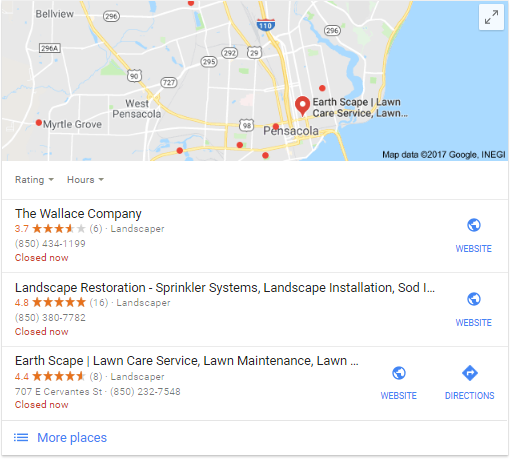The image showcases a detailed map likely from an online service like Google Maps, featuring locations in Florida, specifically areas such as Earthscape Lawn, Pensacola, West Pensacola, Myrtle Grove, and Bellevue. The map is displayed at the top with the characteristic blue water edges representing bodies of water.

Below the map, there are listings of various landscaping companies along with their ratings, contact details, and current status. The first listing is for The Wallace Company, which has a rating of 3.7 stars. This landscaping company’s contact number is 850-434-1199, and it is currently closed. An icon linking to their website is displayed on the right.

The second listing features Landscape Restoration-Sprinkler System, which has a high rating of 4.8 stars based on 16 reviews. They also provide landscape installation services. Their contact number is 850-380-7782, and they are also currently closed.

The final listing is for Earthscape Lawn Care Services, specializing in common lawn maintenance. This company has a rating of 4.4 stars from 8 reviews and is located at 707 East Cervantes Street. Their contact number is 850-282-7548. They are currently closed and offer a website and driving directions.

Each entry is clearly marked with essential details making it easy for anyone looking for landscaping services in these Florida areas.